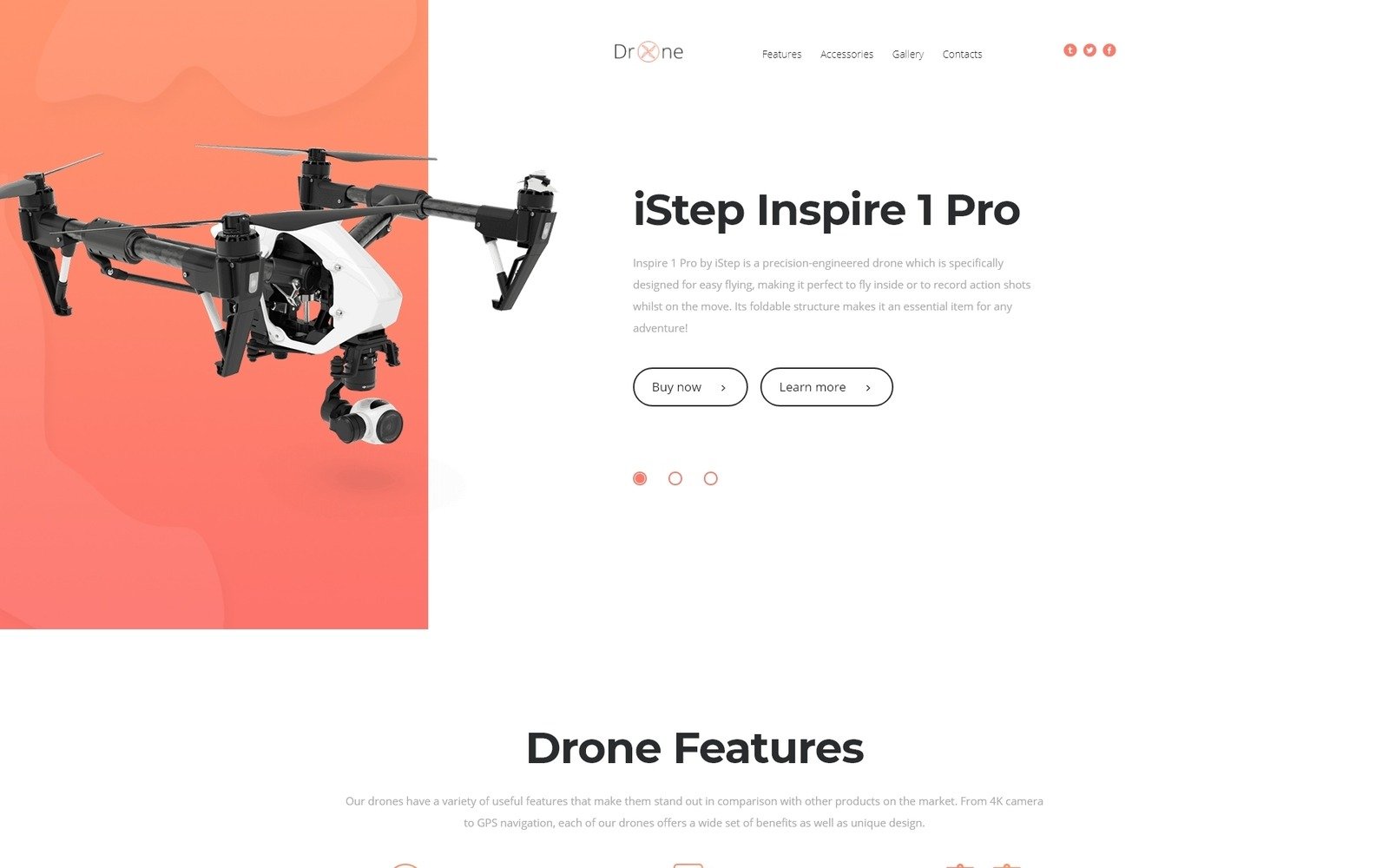A website screenshot showcasing the iStep Inspire 1 Pro drone is presented against an orange background. The white and black drone is positioned on the left side of the image, facing right. At the top of the webpage, the title "drone" is prominently displayed, with a creative "O" designed to resemble a helicopter rotor. The navigation menu includes links to "Features," "Accessories," "Galleries," and "Contacts," alongside social media icons for Tumblr, Twitter, and Facebook.

The iStep Inspire 1 Pro is highlighted as a precision-engineered drone, ideal for both indoor flying and capturing dynamic action shots on the go. Its foldable design makes it a valuable companion for any adventure. Additional buttons labeled "Buy now" and "Learn more" are visible for further interaction.

The text elaborates on the distinctive features of their drones, emphasizing the benefits of a 4K camera and GPS navigation, among other advanced functionalities that set them apart from other market offerings. The image strictly focuses on the drone and the informational content, with no presence of people, animals, birds, plants, trees, automobiles, or bicycles.